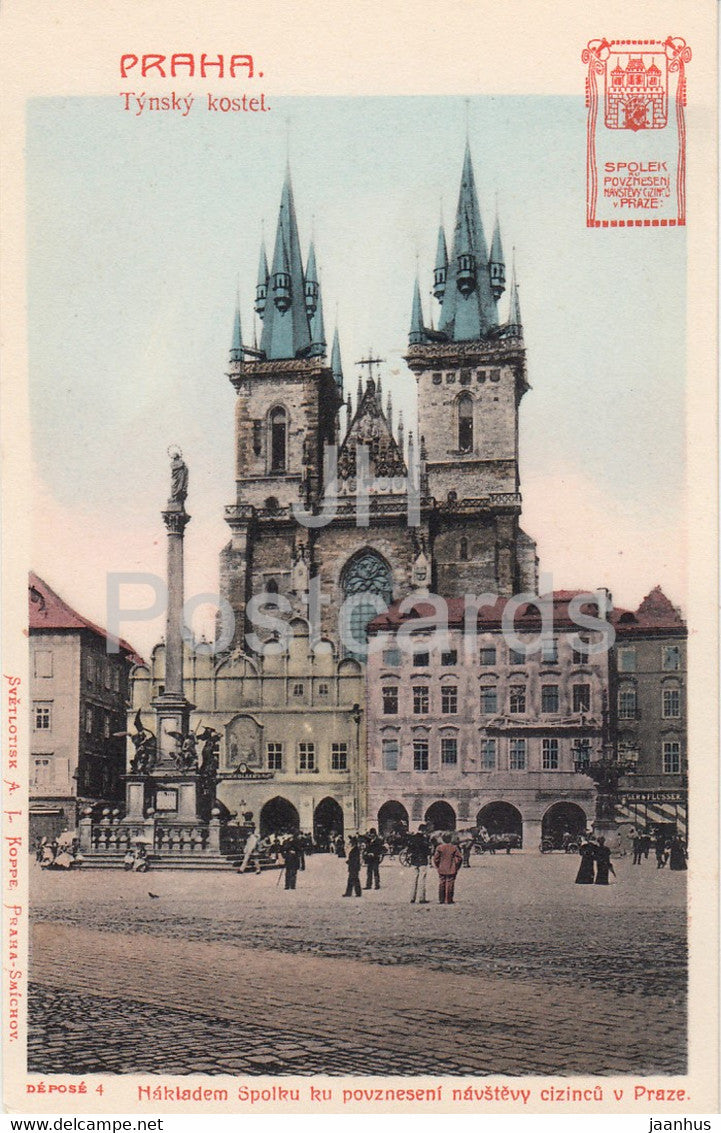This is an old-fashioned, hand-colored postcard from Prague, with the title "Praha Tinsky Kostel" in red at the top left. The postcard is watermarked with "JH Postcards" and features text in a language that appears to be Russian or from Eastern Europe. The prominent building in the image is a grand church with two central towers, each adorned with high, baby-blue pointed roofs. The church features a stained glass centerpiece and sits on an arched base, giving it a stately three-story appearance. In front of the church, there's a spacious cobblestone plaza where several spectators and pedestrians can be seen, some looking up in admiration at the architectural beauty. A tall pillar with a statue, possibly a monument, stands in the courtyard, adding to the historic feel of the scene. The original black and white postcard has been colorized with muted hues of blue, pink, and beige, capturing the old-world charm and vibrant culture of the area.